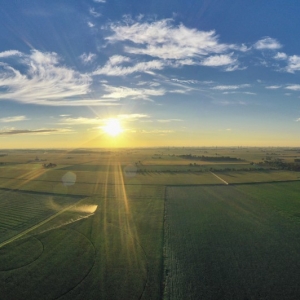This captivating aerial photograph, likely taken from a plane, helicopter, or drone, showcases a stunning sunrise over an expansive agricultural landscape. The horizon is ablaze with shades of orange, transitioning to a clearer blue sky dotted with wispy clouds as it stretches upwards. The scene is meticulously divided with the upper half embodying the vibrant sky, while the lower half is a patchwork of fields and farmlands. In the foreground, a large green field is visible to the right, alongside a pond to the left, and the fields are further segmented by rows of trees and patches of darker brown foliage in the background. The entire landscape is devoid of any structures, vehicles, or people, emphasizing the vast, untamed beauty of rural cultivation. The sunlight cascades dramatically across the scene, casting a warm, yellow hue over the fields, accentuating the cultivated lines left by farm equipment. The image exudes tranquility and the serene, ordered beauty of nature at the break of dawn.